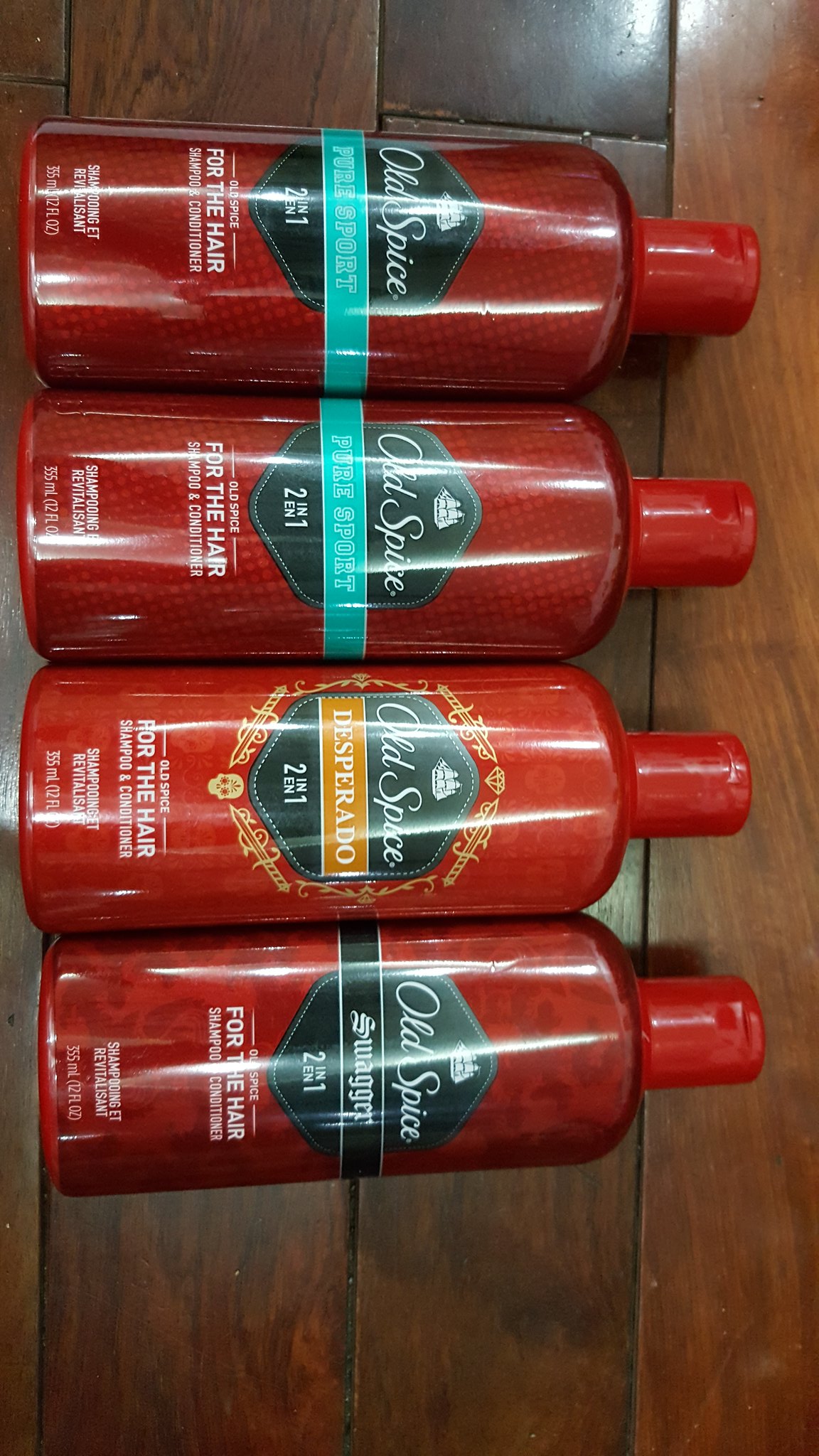The photograph displays four horizontally aligned Old Spice 2-in-1 shampoo and conditioner bottles, laying on a medium to dark brown wooden floor with vertical paneling. All bottles are deep red with slightly lighter red flip-top caps. The branding features the Old Spice cursive logo with diamond-shaped emblems behind it. The first two bottles are labeled "Old Spice Pure Sport 2-in-1," each adorned with an aqua blue rectangular banner. The third bottle reads "Old Spice Desperado 2-in-1" and features an orange banner. The fourth bottle is named "Old Spice Swagger 2-in-1," distinguished by a black rectangular banner. Each bottle clearly states it is for hair care, containing 335 milliliters of product. The arrangement and presentation suggest this image could be used in a sales listing on platforms like eBay, Facebook Marketplace, or Craigslist.